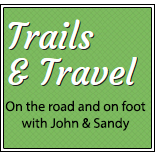This is a detailed graphic image featuring a green square with a distinct white and black border. The green square incorporates a subtle diagonal crosshatch pattern. At the top of the square, large white text reads "Trails and Travels," aligned to the left. Below this, centered text in black states "on the road and on foot with John and Sandy." There are no other images or texts included, making the green box with its textual content the focal point of the design.